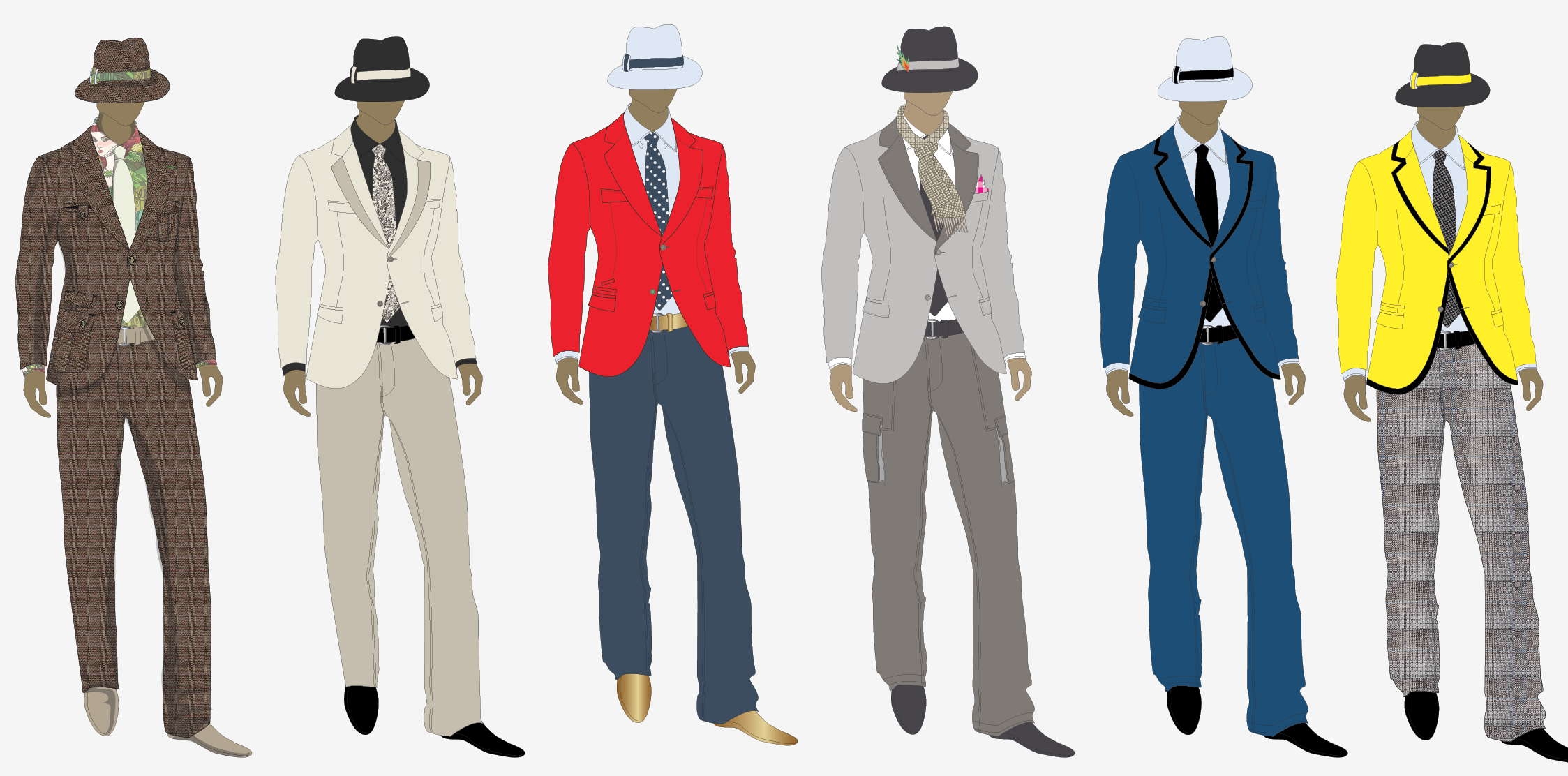The image is a digital drawing oriented in landscape format, featuring six male figures arranged horizontally in a row, each adorned in distinct suits that exhibit various styles and colors. The base mannequins are identical, standing in a subtle, dynamic pose with the right leg slightly raised and the left leg pointed away, all looking vaguely towards the left. Here is a detailed description of each figure's outfit from left to right:

1. **Leftmost Figure:** Dressed in a brown plaid suit with a matching brown fedora. Underneath, he wears a multicolored green shirt paired with a light-colored tie and gray shoes.
   
2. **Second Figure:** Features an off-white jacket and slightly darker ivory-beige pants. He has a black shirt, a black and white patterned tie, and a black hat with a white band, complemented by black shoes.
   
3. **Third Figure:** Sports a striking bright red blazer with dark blue pants. He is wearing a white shirt, a white hat with a blue band, a blue dotted tie, and shiny gold shoes.
   
4. **Fourth Figure:** Adorned in a light gray coat and darker gray pants. His attire is completed with a grayish scarf, gray shoes, and a darker gray hat with a light gray band.
   
5. **Fifth Figure:** Outfitted in a deep blue suit consisting of a blazer and pants. He wears a white shirt, a black tie, a white hat with a black band, and black shoes.
   
6. **Rightmost Figure:** Dons a bright yellow jacket with gray plaid pants, a white shirt, a black hat with a yellow band, a gray tie, and black shoes.

This comprehensive visual showcases six unique designs, each conveying a distinct style through its color, fabric, and accessory choices, forming an intriguing collection of concept men’s suits.